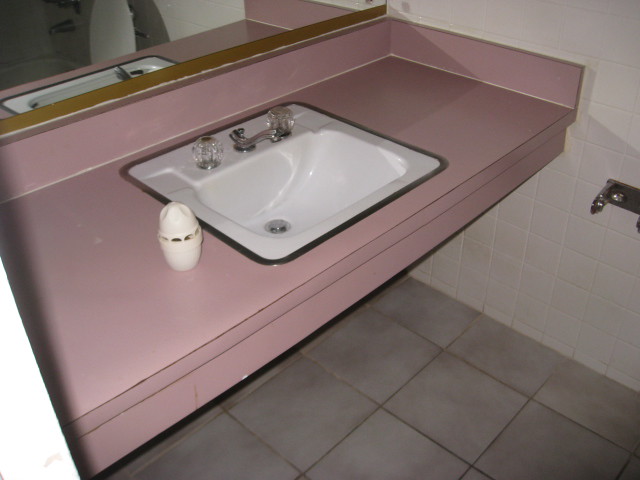This image is a vibrant color photograph taken inside a bathroom. The focal point is a pink counter that extends diagonally from the bottom left corner to the top right of the image, with a subtle under rim for added detail. Centered on the counter is a white porcelain sink, distinctively square with softly curved edges at the corners. The sink is equipped with a sleek stainless steel faucet and drain, flanked by textured plastic knobs for hot and cold water control.

To the left of the sink, just off-center, sits a white air freshener, providing a small touch of freshness to the setting. The sink area is set above a stone floor, featuring square tiles in a sophisticated stone gray color. On the far wall, white tiles provide a clean backdrop, accented by a metal holder mounted on the wall, likely for toilet paper or paper towels.

Above the sink, a mirror reflects not just the sink itself but also various elements of the bathroom behind the photographer. Notably, the bottom left corner of the image is cropped out, possibly due to an object in front of the camera or an overexposed flash that has obscured any detail. This thoughtful arrangement and the interplay of colors and materials create a harmonious and inviting bathroom space.